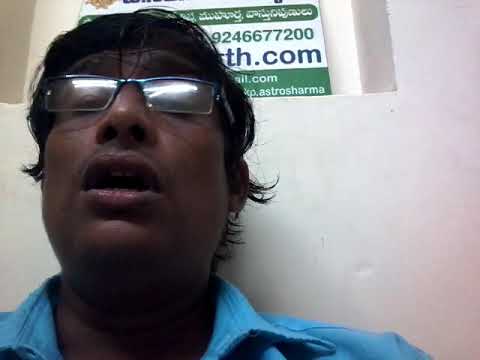The image showcases a close-up view of a man with dark skin and black, medium-length hair, which is slightly curled at the ends. He is positioned on the left side of the photograph, wearing square-shaped glasses and a teal collared shirt. His head is leaning back slightly against a white wall, and he appears to be either asleep or in repose, with his eyes closed and mouth just slightly open, revealing a hint of his upper teeth. The image is taken from an angle that renders his head and shoulders as the primary focus. Above his head, there is a green and white sign embedded in a recessed alcove. Although it's partially obscured, some details on the sign are visible: it includes the phone number "924-667-7200," part of a website "T.H.com," another section "I.L.com," and a name "P. ASTROSHARMA." The setting suggests that the man is in a public place.